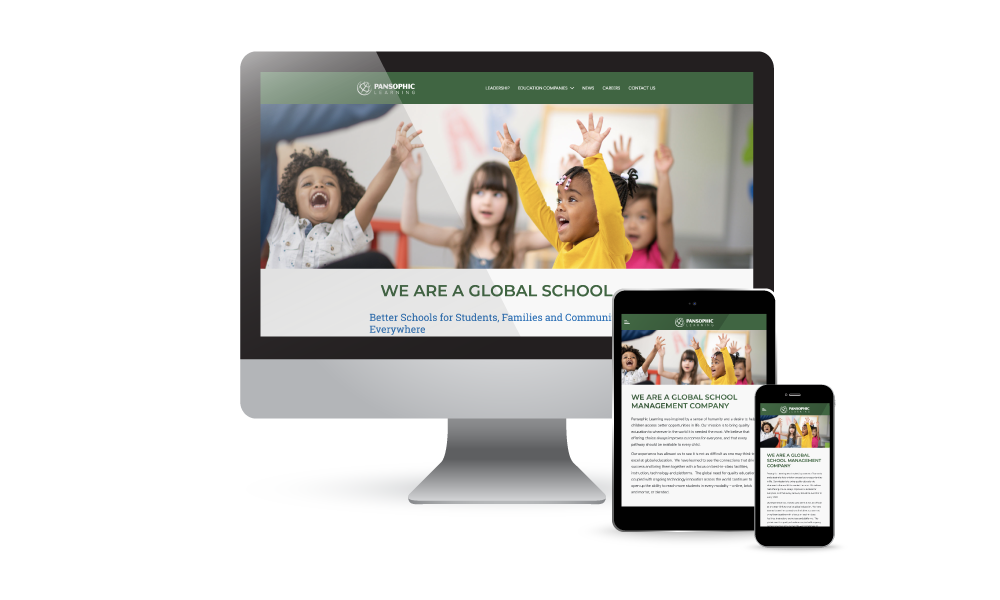An image showcasing the responsive design of a website displayed on a computer monitor, tablet, and smartphone. Each device screen features the same website, with a green navigation bar across the top. On the left side of the bar is a white logo that reads "PENSOFIC." Adjacent to the logo are five navigation buttons. Below the navigation bar, a banner displays an image of four young children, approximately three or four years old, either playing or attending a class, with their hands raised. Underneath the banner, the text "We are a global school" is prominently displayed on a white background. The computer monitor in the image has a gray frame.